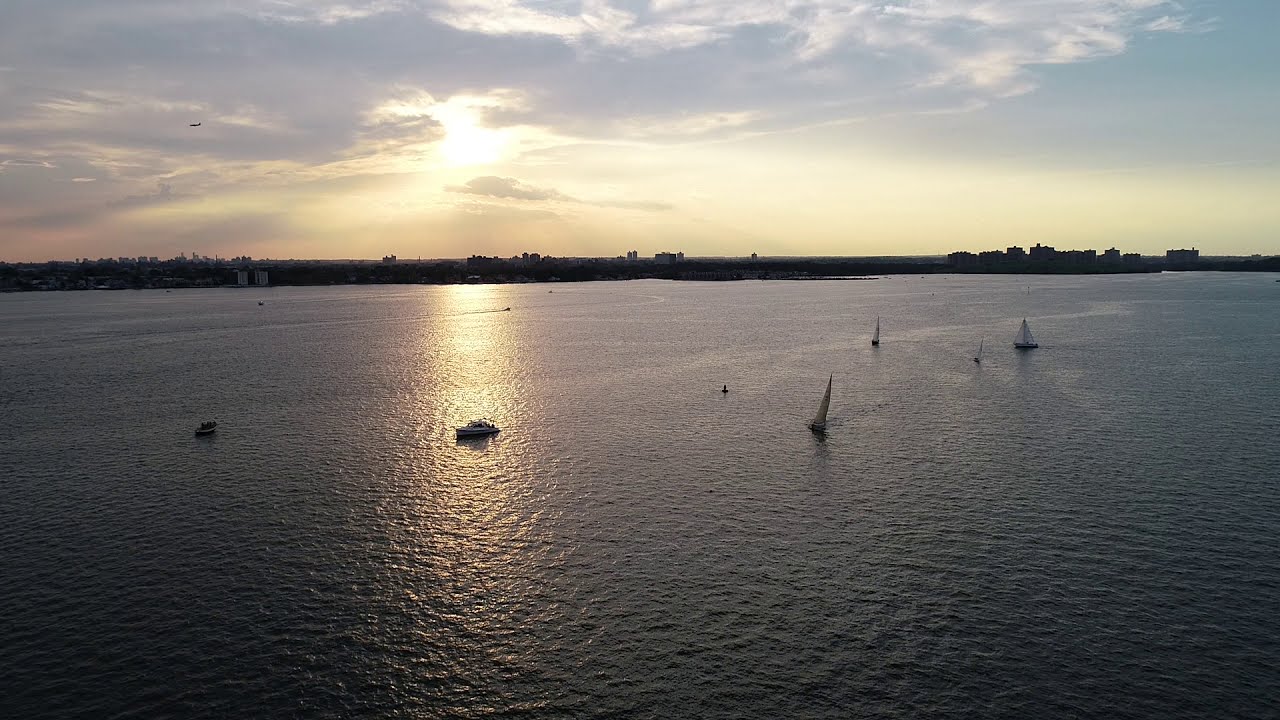The image portrays a serene water scene with a wide, calm expanse of water, possibly a river or sea, depicted in a dark blue or blue-gray hue with small ripples across its surface. The horizon showcases a thin strip of land peppered with tiny buildings, appearing almost like a silhouette against the complicated transition of light and shadow. Above, the sky is predominantly cloudy, with the sun partially obscured but casting a yellowish glow through the gaps and reflecting subtly on the water below. In the water, several boats, including sailboats, are scattered, some coasting gently, adding a touch of life to the tranquil setting. The overall ambiance suggests either late afternoon or a particularly overcast day, with the interplay of light giving the scene a peaceful, almost dreamlike quality.